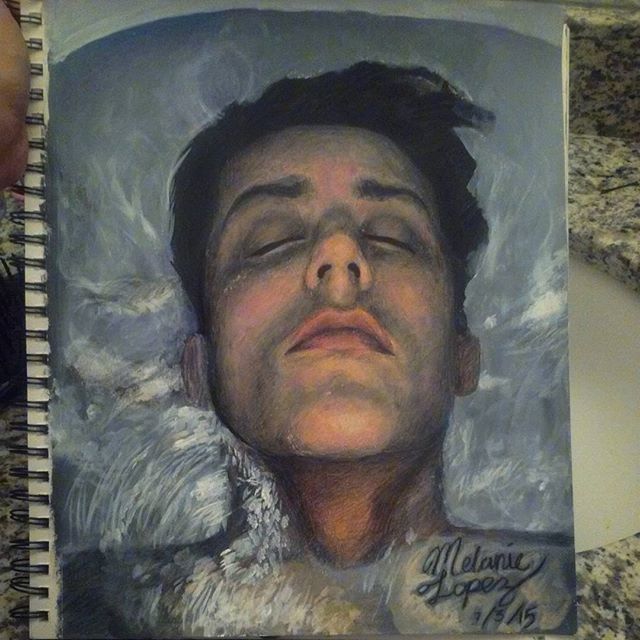The detailed sketch depicts a male figure with closed eyes, seemingly enveloped in rushing water. His head, adorned with black hair, is the focal point of the drawing, with only a hint of his shoulders visible. The gray-toned water, which is unusual in its color choice, contrasts with the typical blue and appears to be cascading around him, giving the impression of floating or being submerged. The sketch is drawn on a sketch pad, partially shown against a background that appears to be a marble surface, potentially a tabletop or sink counter. The artist's signature, "Melanie Lopez," and the date "1-3-15" are evident at the bottom of the page, adding a personal touch to the intriguing and emotive artwork.